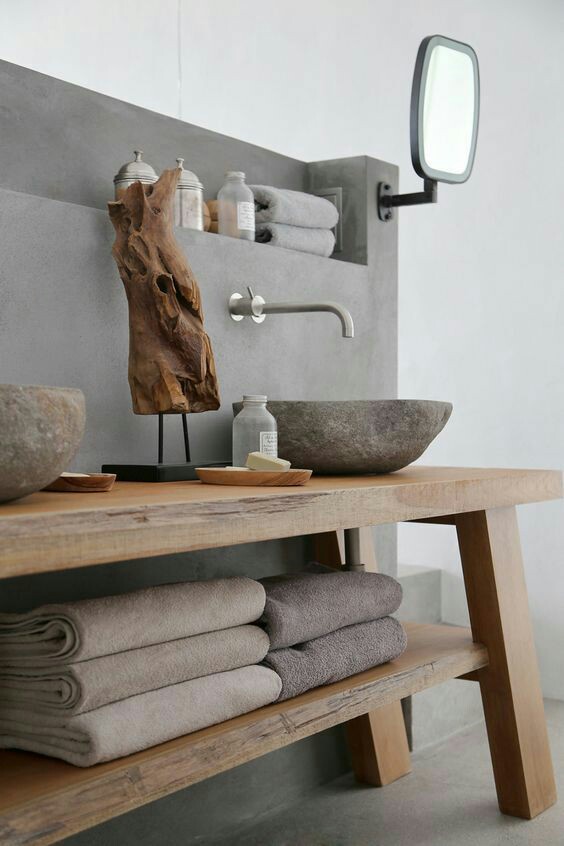This color photograph showcases a minimalist-style bathroom with a calm and uncluttered aesthetic. Dominating the scene is a simple wooden bench, possibly made from untreated wood, exuding a natural charm. This bench features a convenient lower shelf where five neatly folded towels rest; three are a light gray hue, while the remaining two are a darker shade of gray.

Atop the bench sits a large, shallow gray bowl that functions as the sink. This unconventional sink is complemented by a wall-mounted, unpolished gray faucet, which blends seamlessly into the gray backdrop. Above the faucet, a small shelf holds a couple of gray towels and three clear bottles, adding to the bathroom’s cohesive design.

To the right of the sink on the bench, there is a large bottle accompanied by a small, intriguing sculpture in an orangish color, lending a touch of warmth and personality to the serene setting. The overall effect is one of understated elegance, where every element is thoughtfully curated to maintain the minimalist theme.